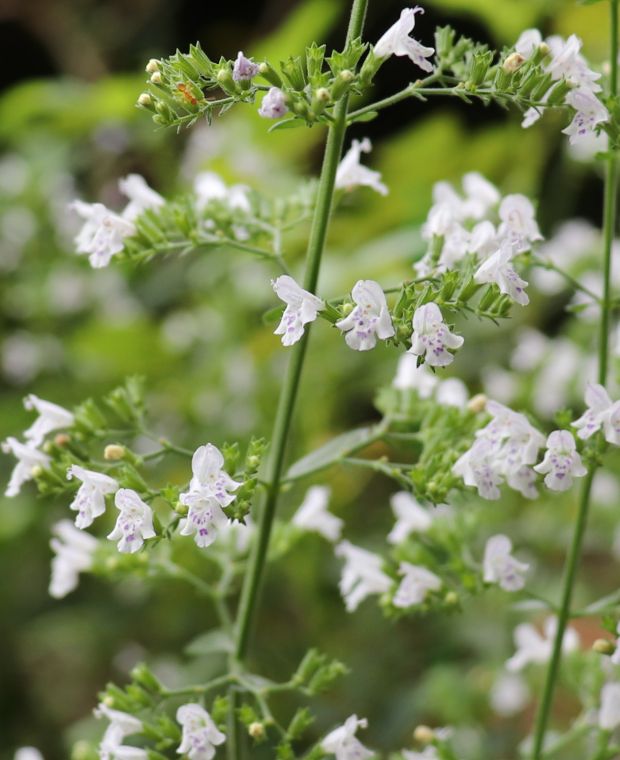The image showcases two distinct stems of a plant, rising from the bottom to the top of the frame, prominently situated near the right edge. The stems are green and support an array of small, delicate flowers, predominantly white with hints of purple. Several buds are also visible, still unopened and green. The surrounding leaves are green, adding to the plant's lush appearance. The background is a blurry expanse of green, indicating other plants with large leaves, but it remains indistinct due to the focus being on the main plant. The overall scene suggests a bright, possibly sunny day, highlighting the natural beauty and serenity of this blooming field.